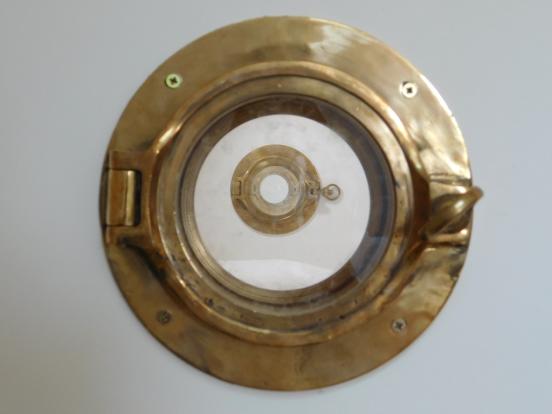The image showcases a brass or copper-colored circular metal object against a gray background, without a border. The circular item features a cutout in the center, encircling another smaller circular element with a white middle. The larger brass ring has a darker copper-colored ring around the central white space. The object is mounted with a hinge on the left and a knob or key-like handle on the right, suggesting it can be opened by turning the knob to pivot left on the hinge. The ring is secured with four screws, two at the top and two at the bottom. Inside the central cutout, there appears to be a small photograph or depiction of the circle itself, maintaining the metallic, copper tone consistent with the outer ring. The object’s detailed craftsmanship and intricate parts make it a striking focal point in the image.